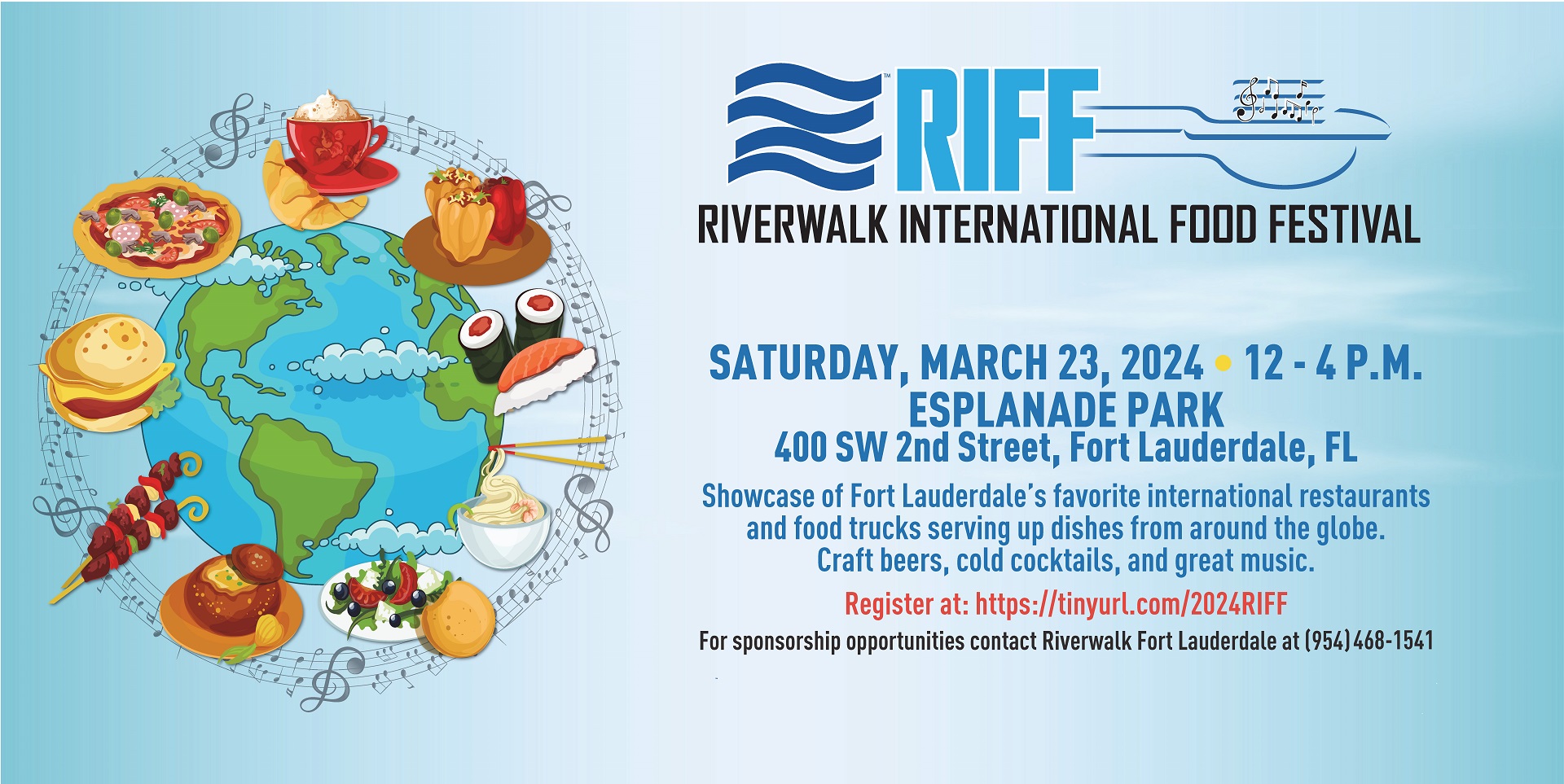This vibrant poster advertises the Riverwalk International Food Festival. Dominated by hues of blue, the top of the poster displays large blue letters "R-I-F-F" with dark blue wave designs beside it, symbolizing the Riverwalk. To enhance the nautical theme, the letters resemble the deck of a boat. Below, in blue font, the festival details are clearly stated: "Saturday, March 23, 2024, 12 to 4 p.m. Esplanade Park, 400 SW 2nd Street, Fort Lauderdale, Florida." 

A striking red link urges attendees to register, with further information about sponsorship opportunities available through contact at 254-468-1541. On the left, a vibrant globe illustration in green and blue is encircled by a variety of international foods such as sushi, pizza, a hamburger, a croissant, stuffed peppers, a frothy drink, shish kebabs, and a bread bowl. These dishes are interspersed with musical notes, evoking a celebration of global cuisines and entertainment. The colorful design against a sky-blue background effectively captures the festive spirit of the event.